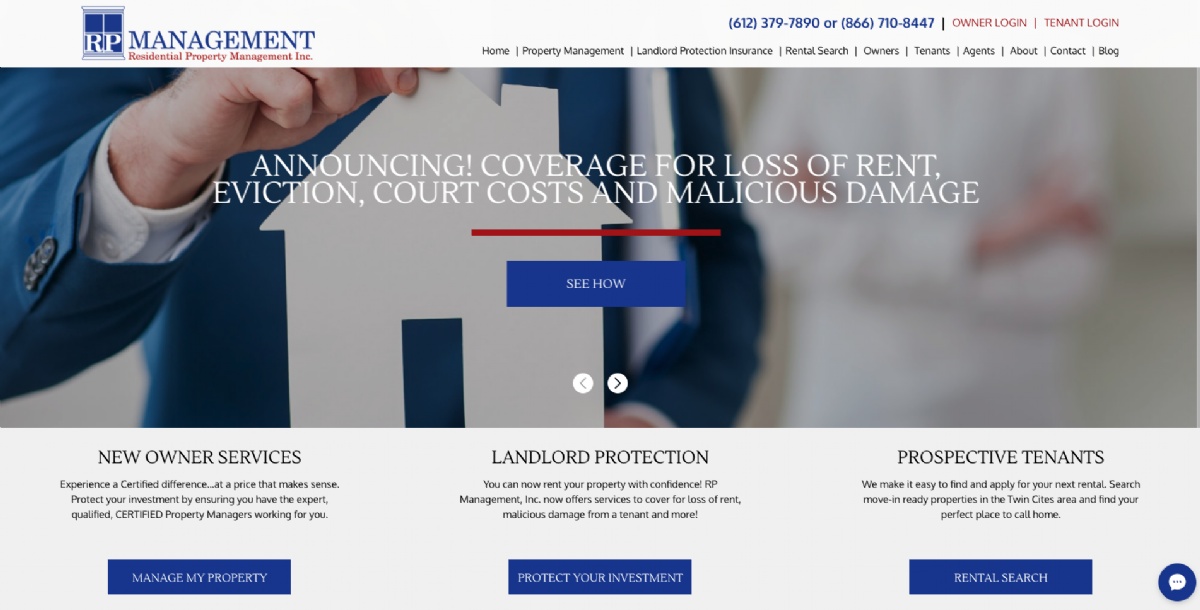This image depicts a detailed screenshot of a website for RP Management, Residential Property Management Incorporated. Dominating the background is an image featuring a cropped view of a woman dressed in a blue suit with a white shirt underneath, holding a small paper cutout of a house. 

Overlaid on the image in bold, white text is an announcement that reads: "ANNOUNCING COVERAGE FOR LOSS OF RENT, EVICTION, COURT COSTS, AND MALICIOUS DAMAGE." Just below this proclamation is a prominent blue button labeled "See How."

At the top of the screen, the website's header contains the RP Management logo and name, along with their contact phone number. Adjacent to this are two text links for users to log in, one for owners and one for tenants.

A navigation bar beneath the header includes links to various sections of the website: Home, Property Management, Landlord Protection Insurance, Rental Search, Owners, Tenants, Agents, About, Contact, and Vlog.

The footer of the page presents three additional buttons that direct users to unspecified areas. Finally, in the bottom right corner, there's a blue circle with a white speech bubble icon, indicating the presence of a chat bot for user assistance.